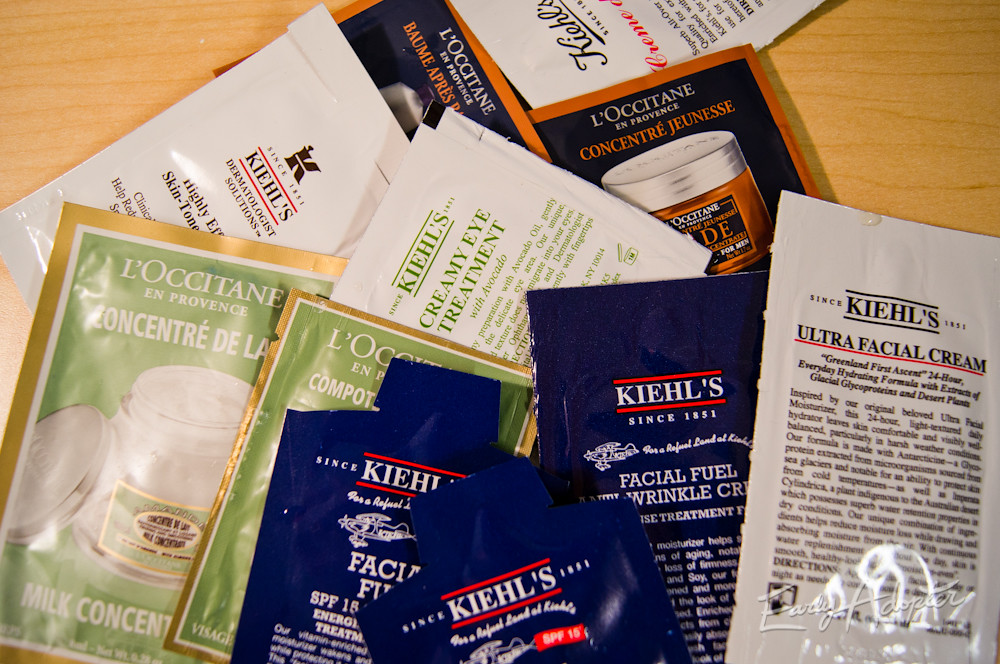A collection of skincare product samples is spread out on a beige wooden table, illuminated by a touch of sunlight. The assortment includes Kiehl's Ultra Facial Cream in a white packet, Kiehl's Facial Fuel Anti-Wrinkle Cream in a blue packet, and Kiehl's Creamy Eye Treatment in a white packet adorned with green text. Additionally, there is a packet of L'Occitane Milk Concentrate, distinguished by its green packaging and gold border. Sun flares from the camera lens add a warm glow to the scene, enhancing the inviting presentation of these premium skincare products.